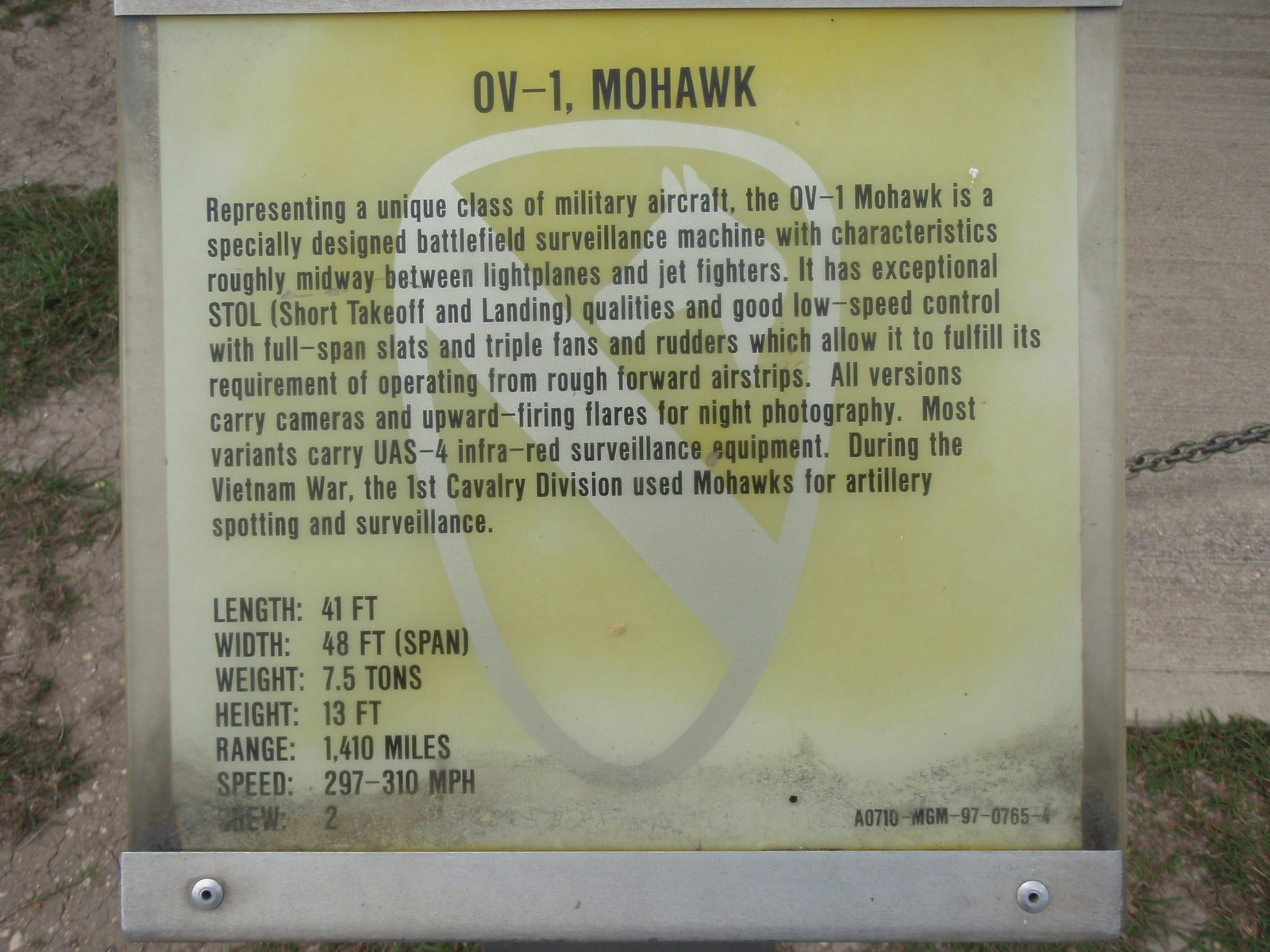The photo was taken outside and predominantly features a laminated sign held in a metal stand. In the background, there is a mixture of green grass and dirt, a concrete road, and a metal chain. The sign has a yellow background and includes detailed information about the OV-1 Mohawk, a unique class of military aircraft designed for battlefield surveillance. The sign begins with "OV-1 Mohawk" and describes the aircraft's capabilities, including its exceptional stall, short takeoff and landing qualities, good low-speed control with full span slats, and triple fins and rudders that enable it to operate from rough forward airstrips. It also mentions the aircraft's use in the Vietnam War by the 1st Cavalry Division for artillery spotting and surveillance. The bottom of the sign lists the aircraft's dimensions, including length, width, height, weight, range, speed, and crew details. A white shield with a horse is displayed in the top right corner of the sign.